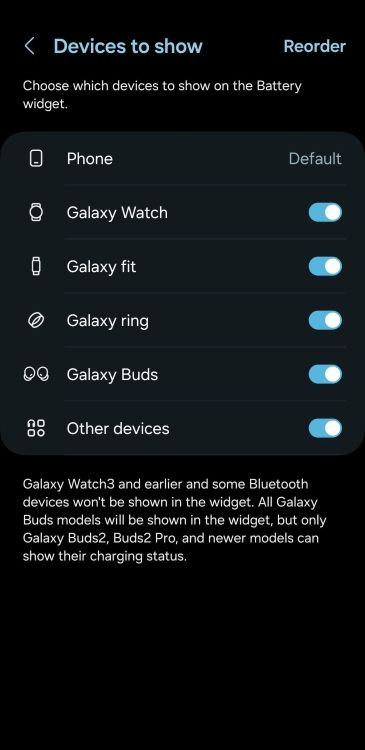Screenshot from an Android device highlighting the "Devices to Show" settings page. At the top, there is a back arrow and a title, "Devices to Show," with a bold subtitle, "Reorder." Below the subtitle, an instruction reads, "Choose which devices to show on the battery widget."

The list of devices includes:
1. **Phone** (default)
2. **Galaxy Watch**
3. **Galaxy Fit**
4. **Galaxy Ring**
5. **Galaxy Buds**

Each device has a toggle switch set to "on," indicated by a blue switch. This suggests they are all connected via Bluetooth. A note at the bottom states, "Galaxy Watch 3 and earlier and some Bluetooth devices won't be shown in the widget. All Galaxy Buds models will be shown in the widget, but only Galaxy Buds 2, Buds 2 Pro and newer models can show their charging status."

The background of the screenshot is black with white text in a mellow font, accented by blue toggles.